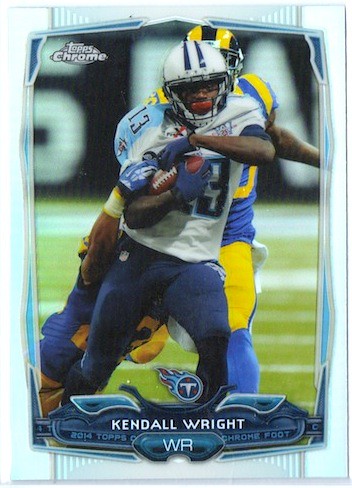This detailed image appears to be a cropped photograph of a card from a mobile screen or a game console, portraying American football players from a 2014 Topps Chrome card. The central figure, an African-American player named Kendall Wright, is seen running with a football, wearing a white jersey with the blue number 13 and blue pants. Surrounding him are two more African-American football players; one in the foreground is clad in a yellow and blue uniform attempting to tackle Wright, while another player, mostly obscured, is visible in the background. Both wear similar yellow and blue gear, indicating they are likely teammates. The players are donned in helmets, knee guards, gloves, and chest pads. The card features vibrant colors including green, white, yellow, blue, black, brown, and shades of navy blue. Texts at the top left and bottom sections of the card read "Topps Chrome" and "Kendall Wright, WR," respectively, along with a team logo and symbol.